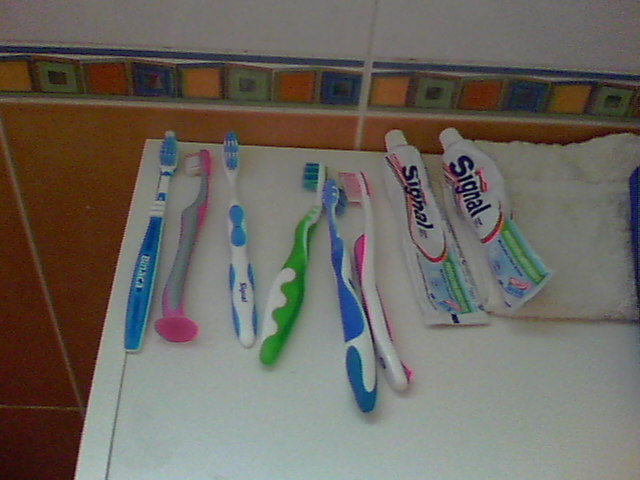The photo captures a detailed scene of a bathroom countertop, focusing on an array of toothbrushes and toothpaste. The white counter hosts six manual toothbrushes and two slightly crumpled tubes of Signal toothpaste. From left to right, the toothbrushes are colorfully diverse: the first is blue and white, followed by a pink and gray children's toothbrush with a suction stand, then another blue and white one, a green and white one, a darker blue and white one, and finally a hot pink and white toothbrush. Additionally, a white hand towel is positioned on the far right. 

The background wall displays a distinctive tile pattern: white tiles at the top, followed by a decorative strip of small mosaic-like tiles featuring a sequence of colors including yellow, avocado green with a blue square inside, orangey-red, and blue with an indistinguishable center color. Below this ornate strip, the tiles shift to a light reddish-brown hue. This intricate background complements the orderly arrangement of dental hygiene items on the counter.